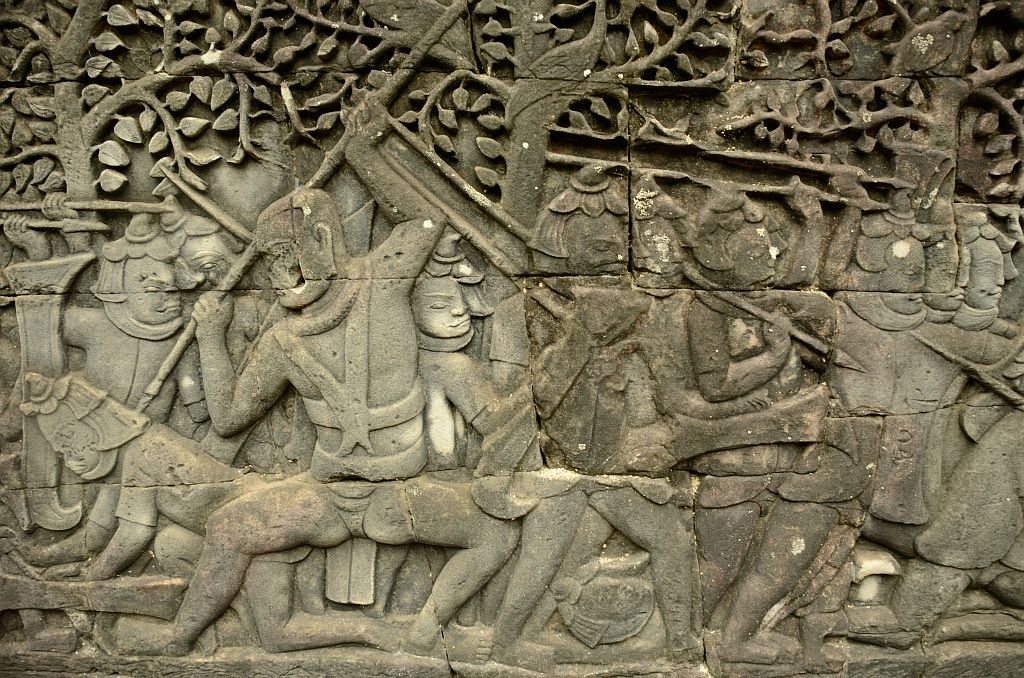This horizontally aligned rectangular image depicts an ancient stone artwork that portrays a group of tribal warriors. The stonework appears worn with a predominant gray color and touches of brown in the center and top. The scene is a close-up shot, providing intricate details of the crafted figures and surrounding elements. The upper portion of the artwork features carved trees with leaves adorning branches that stretch in various directions. Below, a number of nearly unclothed men are engaged in battle; they wield spears, some of which are raised aggressively. On the left, a warrior squats facing the viewer but glances over his right shoulder, a spear held above his head. Another warrior stands behind him with closed eyes. Additional figures are partially visible, overlapping each other, contributing to the densely packed composition. The right side of the scene shows a couple of figures walking calmly with spears over their shoulders, seemingly detached from the conflict. Notably, none of the figures are depicted wearing shoes. The detailed craftsmanship and stylistic elements suggest an ancient origin, reminiscent of historical or possibly Egyptian artwork.